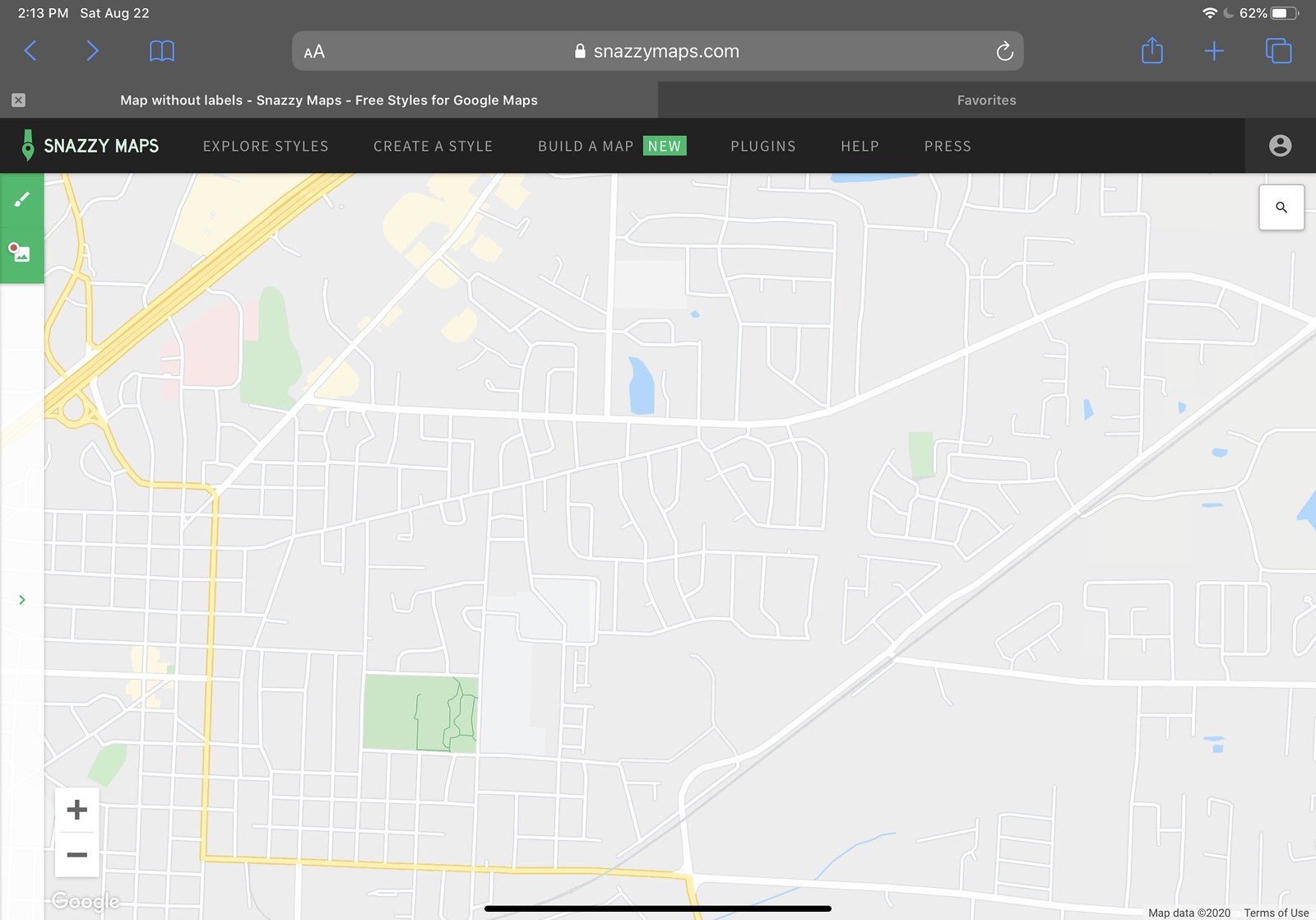The screenshot, captured on an Apple device, displays the Safari browser at 2:13 PM on August 22nd. The device shows a full Wi-Fi signal, is in Do Not Disturb mode, and has a 62% battery level without charging. The active website is snazzymaps.com, with two tabs open: one for the map and another for favorites. The Snazzy Maps interface highlights options such as "Explore Styles," "Create a Style," "Build a Map" (a new feature), "Plugins," "Help," and "Press." In the upper right corner, there's a clickable option to view the user’s Snazzy Maps profile. The displayed map, devoid of labels, features various small subdivisions and is intersected by solid white and yellow lines, particularly noticeable in the upper left corner.